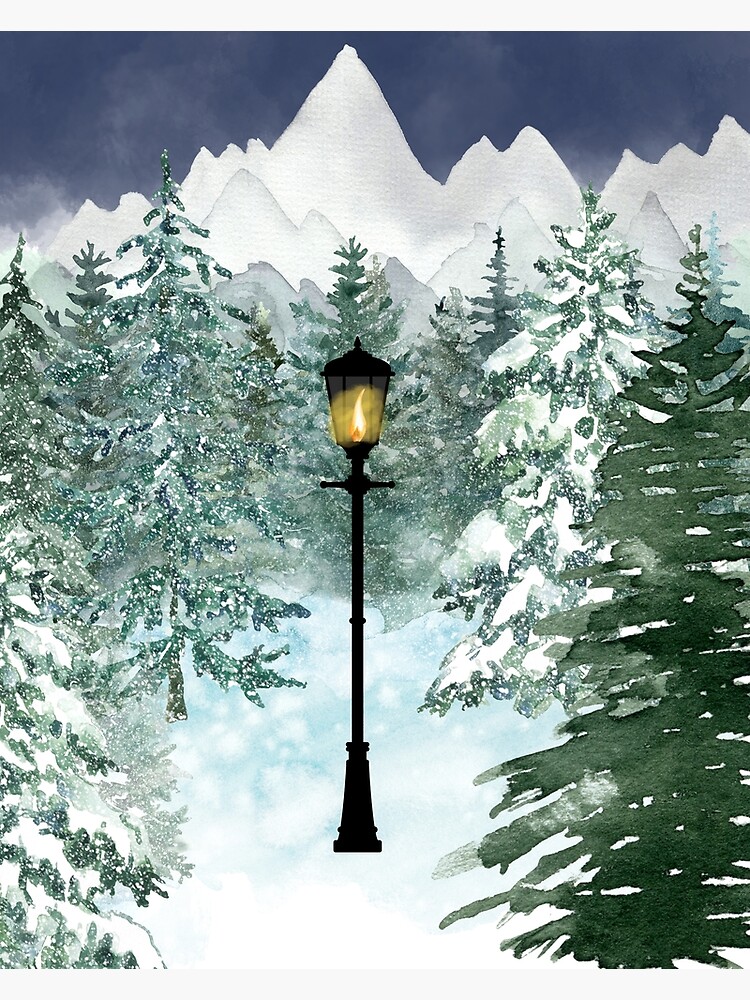This impressionistic painting captures a serene winter scene with an artistic blend of media, possibly watercolor. In the foreground, a black lamppost stands prominently in the center, surrounded by an array of tall evergreen trees, some of which are heavily blanketed in snow. The lamppost, featuring a small cone at the base and a long body leading up to a cross piece, supports a glowing lamp with angled glass panels, radiating a warm yellow and orange flame with a black cap above it. The ground around the lamppost is adorned with white and blue dabs, mimicking the look of freshly fallen snow. Encircling this central element, the evergreen trees create a protective ring, their varied shades of green highlighted by the snow, which gives a watercolor effect. Beyond this secluded scene, towering white mountains rise steeply in the background, with subtle gray outlines distinguishing the different layers of peaks. Above, the sky transitions from a dark blue to a light gray, creating a sense of depth and the presence of distant fog, enhancing the atmospheric feel of a snowy landscape, perhaps in the midst of a peaceful snowstorm.